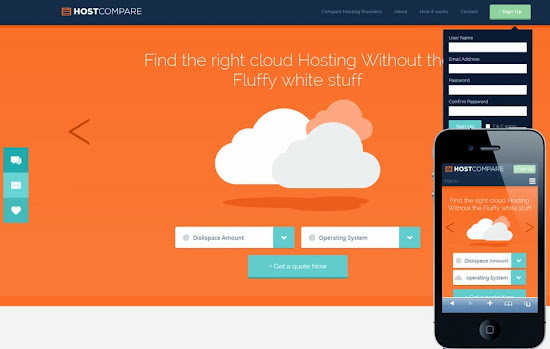**Caption:**

A vibrant and visually engaging webpage from Host Compare is displayed, with an orange background that sets a lively tone. The header reads, "Find the right cloud hosting without the fluffy white stuff," emphasizing no-nonsense service. Three clouds of varying colors — one pure white, one grayish, and one orange blending into the background — highlight the theme. Below, a dark orange puddle adds a splash of color.

Interactive dropdown menus allow users to customize their search based on storage space and operating systems. A prominent green button invites users to "Get a Quote Now." On the left-hand side, a form in black and white neatly asks for personal information, like name and other details.

Next to the form, an image of an iPhone shows a mobile-friendly version of the app. The app interface is described, featuring two side-by-side boxes and a third green box centered below for getting a quote. Each element is meticulously aligned, ensuring clarity and ease of navigation.